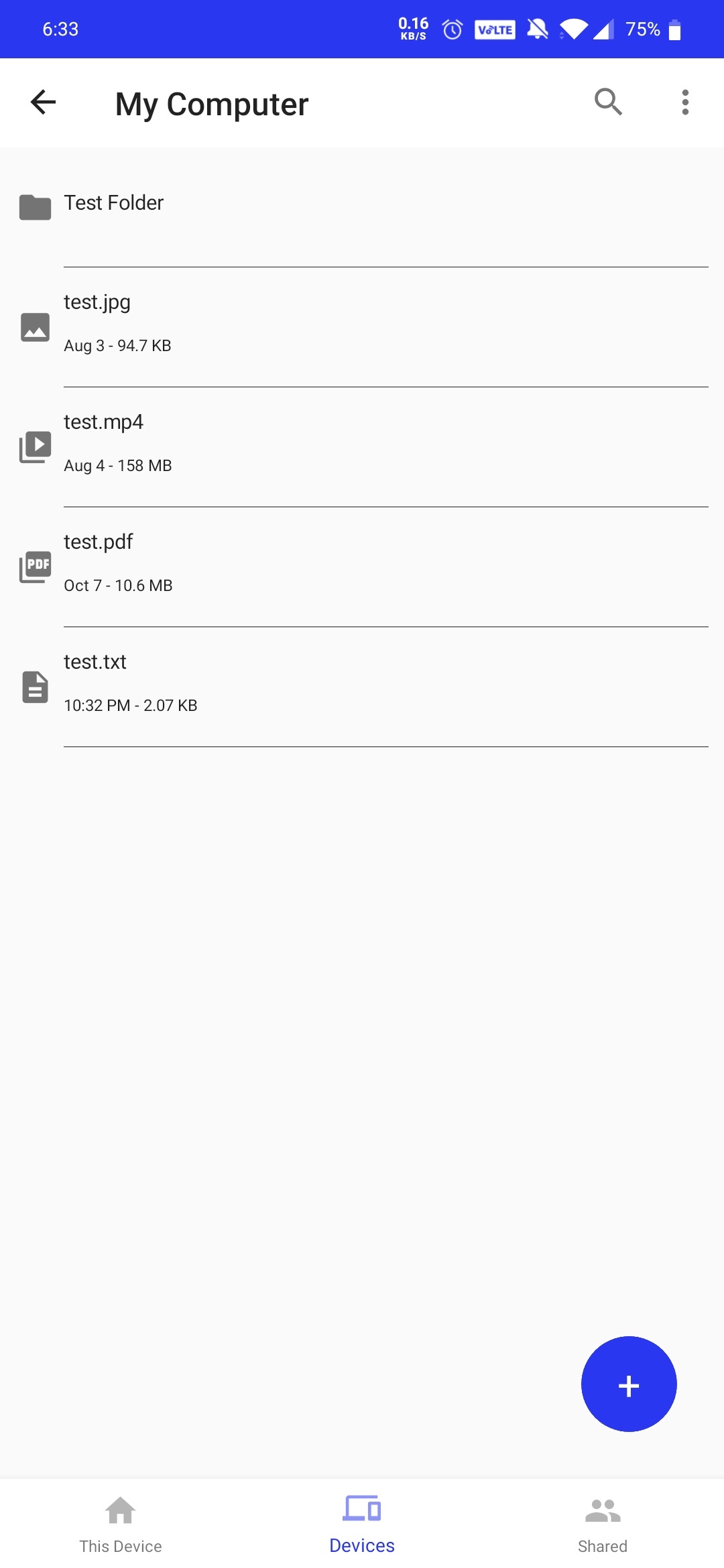In this image with a light gray background, several items and icons are displayed, each providing distinct pieces of information. At the top, there is a numerical display reading "633" for the count labeled "Tom," a battery icon showing "78%," and the numbers "76" and "78." Adjacent to these is a left arrow, likely indicating a back function, followed by icons for a magnifying glass (typically representing search) and three vertical dots (often indicative of a settings or options menu).

Below, there is a "test" folder icon resembling a traditional file folder. Inside this folder, several files are listed with relevant icons and details:
1. **test.jpg** - This is accompanied by an image icon and is listed with a date of August 3rd and a file size of 94.7 kilobytes (KB).
2. **test.mp4** - Accompanied by a video icon (a square with a triangle pointing to the right), it is dated August 4th and has a file size of 158 megabytes (MB).
3. **test.pdf** - Associated with a PDF icon, it is dated October 7th and has a file size of 10.5 MB.
4. **test.txt** - Displayed with an icon resembling a sheet of paper with two lines indicating text, it is time-marked at 10:32 PM and has a file size of 207 KB.

At the bottom right of the image, a blue square with a white plus sign is visible, presumably for adding new items. Below this, navigation options labeled "this device," "devices," and "shared" are listed, indicating different available sections or categories in the interface.